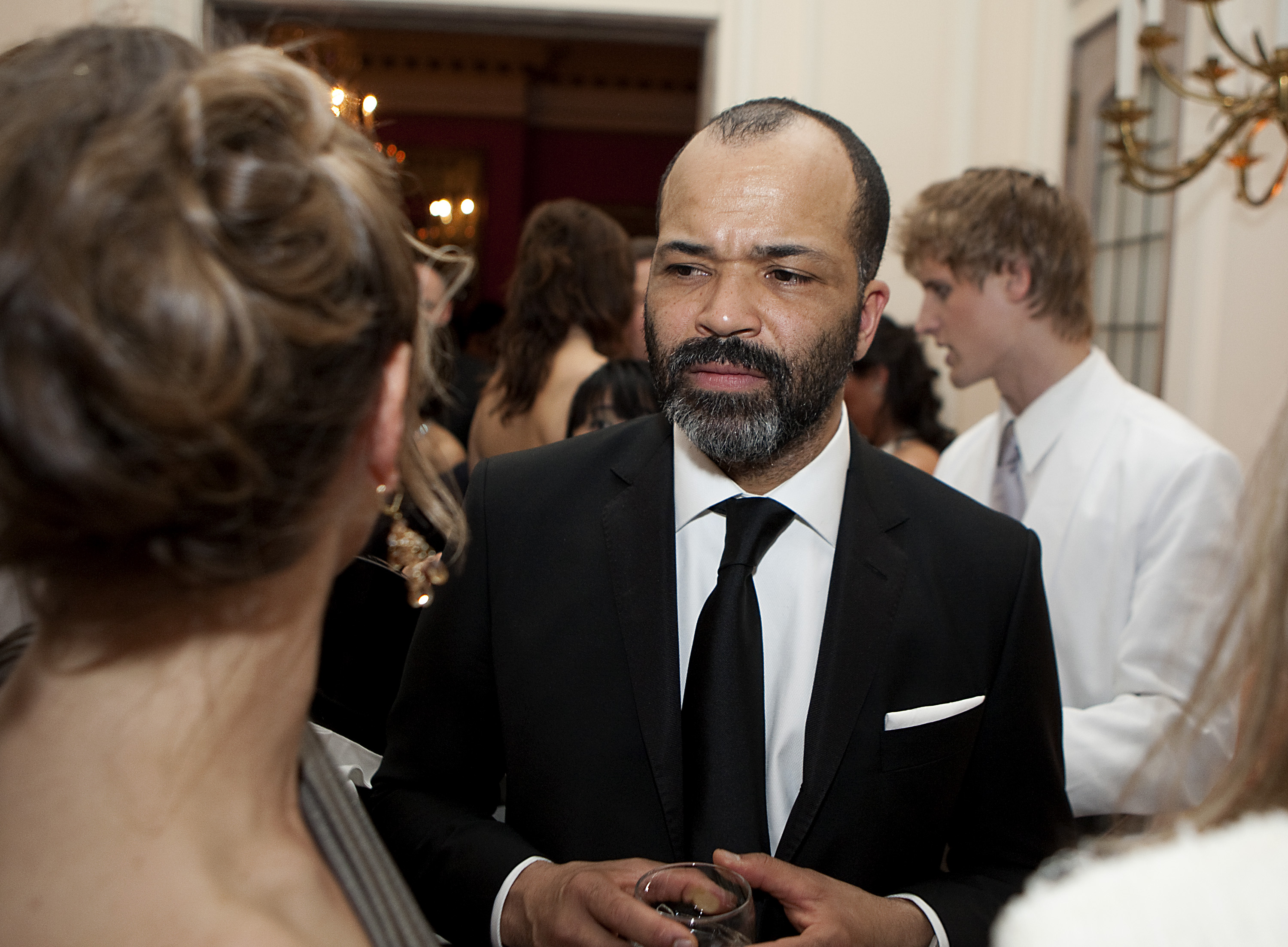In this photograph, the central figure is a middle-aged African-American man, possibly in his mid-50s, dressed in formal attire. He is wearing a black business jacket punctuated with a white handkerchief in the front pocket, a neatly buttoned white dress shirt, and a solid black tie. His appearance is distinctive with a partially bald head and short-cropped hair, accented by a beard and mustache speckled with patches of gray and white. 

The man, who resembles actor Jeffrey Wright, is holding a wine glass in both hands and appears to be in a thoughtful or focused conversation. His brow is slightly furrowed, suggesting concentration or perhaps mild confusion. To his left, a woman in a gray evening gown with gold dangling earrings and her hair styled in a bun, is facing him, although only the back of her head is visible. Additional people fill the background, engaged in their own conversations, contributing to the bustling, social atmosphere of what seems to be a formal event or party. The scene captures a candid moment amid the elegance, with chandeliers and other opulent decorations enhancing the sophisticated setting.